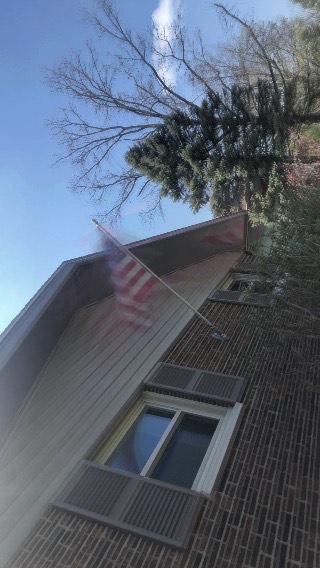This image, taken at an angle with the picture turned on its side, features the side of a brown brick house characterized by dark brown shutters and ecru window frames and trims. Dominating the scene is an American flag attached to the house, fluttering in the breeze. The roof, though primarily viewed from the underside due to the angle, appears to be trimmed with light brown wood paneling. Below one of the large, side windows with its silver trim are some bushes, while a barren tree and a tall conifer stand prominently against the bright, blue sky. White clouds dot the sky, and the overall photo, likely an older image, appears somewhat desaturated yet depicts a clear, sunny day with vivid daylight illuminating the house and its surroundings.